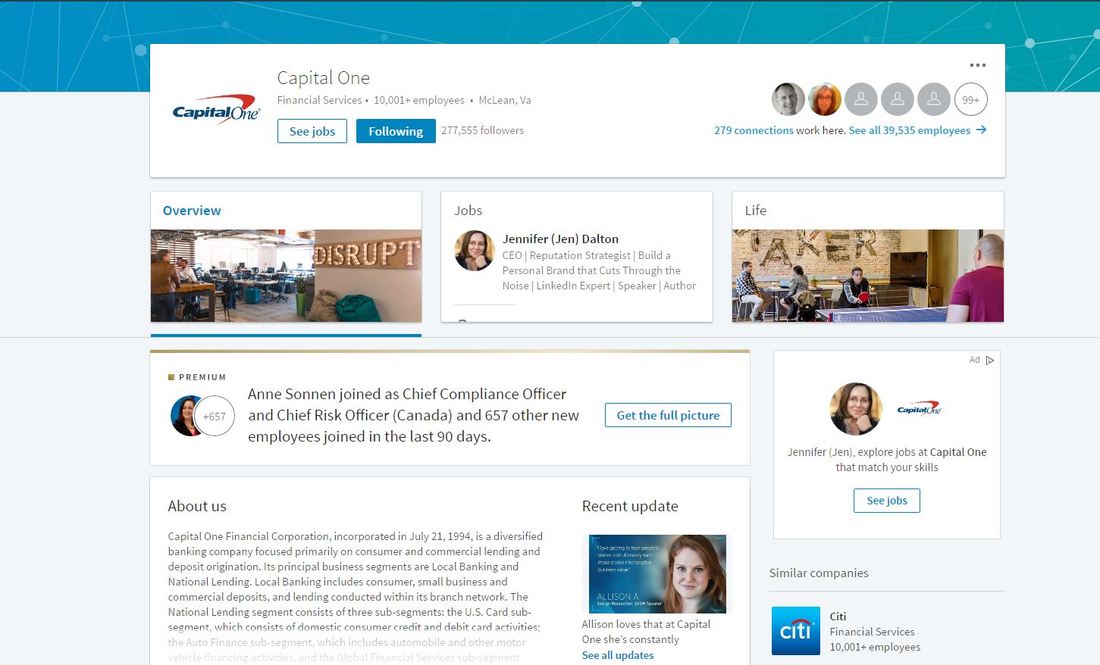The image features a detailed overview of Capital One's LinkedIn page. In the top left corner, "Capital One" is prominently displayed in blue with a red switch icon next to it. To the right, "Capital One Financial Services, 10001+ Employees, McLean VA" is printed alongside two buttons: "See Jobs" in white and "Following" in blue, indicating that the page has 277,555 followers.

In the top right section, it is noted that "279 connections work here" and a link to "see all 39,535 employees" is available. The bottom section is divided into several parts: 

- **Left Side**: An "Overview" tab is visible, along with "About Us" text detailing Capital One Financial Corporation’s incorporation on July 21, 1994, and a description of its focus on consumer and commercial lending, deposit origination, and business segments, though the full text isn't visible.

- **Right Side**: Tabs labeled "Jobs" and "Life" are highlighted. A specific mention is made of Jennifer Jen, Delta, described as a CEO, reputation strategist, LinkedIn expert, speaker, and author.

- **Center Left**: A "Premium" section notes Arne Sonnen’s recent appointment as Chief Compliance Officer and Chief Risk Officer of Canada, along with the addition of 657 new employees in the last 90 days. A blue button labeled "Get Full Picture" is present for more information.

- **Right Center**: An advertisement encourages users to explore job opportunities at Capital One, with a blue "See Jobs" button.

- **Bottom Left**: The "About Us" section continues to detail Capital One's diversified banking services, but the full text isn't completely visible.

- **Bottom Right**: A "Recent Update" mentions Alison's positive experience at Capital One with a link to "See All Updates" in blue. Additionally, there's a "Similar Companies" section listing CT Financial Services with 1001+ employees. 

This elaborate LinkedIn page layout provides a comprehensive insight into Capital One's corporate details, job opportunities, and recent updates.